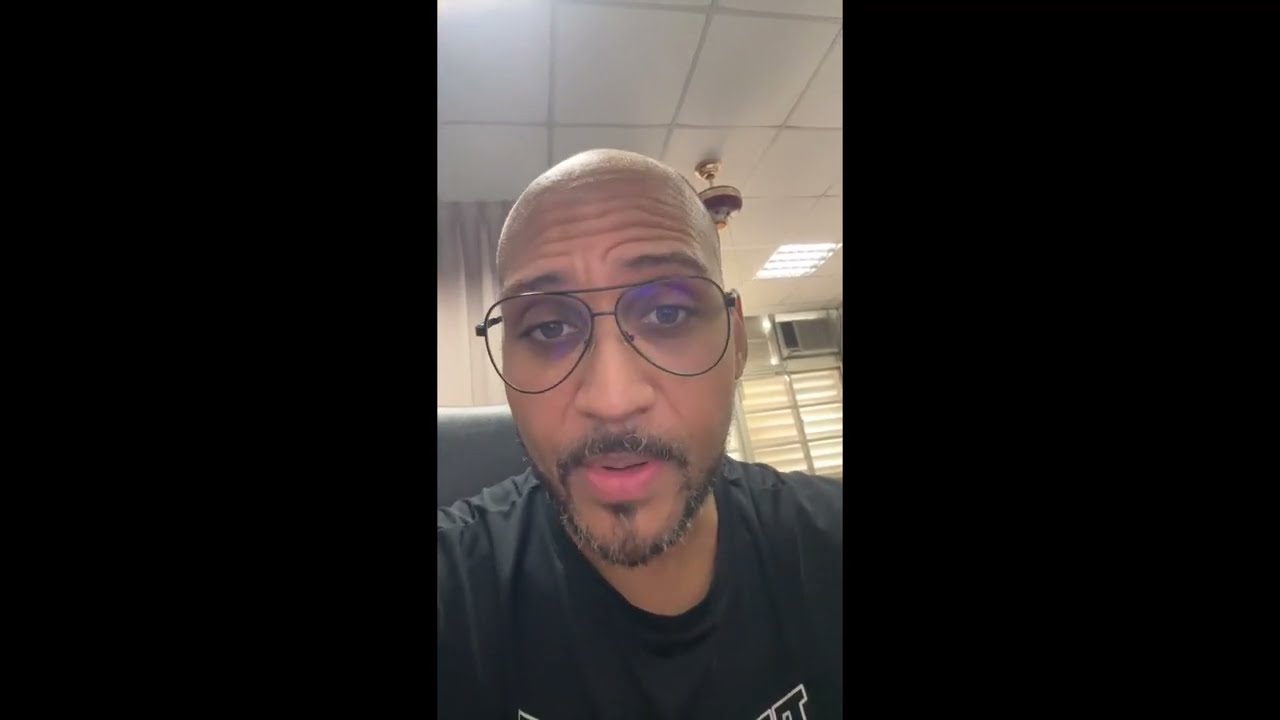The image features a vertical strip at the center flanked by 2-inch wide black bars on both sides. The central photo, approximately 2 inches wide and 1.5 inches tall, showcases a close-up of a middle-aged bald black man wearing oval-shaped, thin-rimmed glasses that appear oversized for his face. He has a short mustache, a goatee, and a chin strap beard, all of which are black. His expression is intense, staring directly into the camera with a slightly furrowed brow, and he appears to be speaking. His lips are red, with the bottom lip more prominent. The man is wearing a black t-shirt, though the text on it is partially cut off. Behind him, the room features white ceiling panels with an embedded light fixture, a window on the right side blocked by shutters, an air conditioning unit set among glass blocks allowing some daylight through, and a set of white curtains. There is also a gold stand with a circular base in the background, adding to the detailed setting of the image.